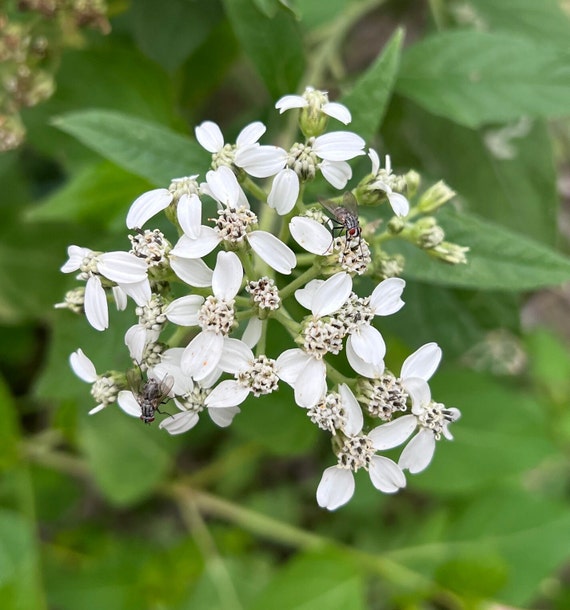This image is a close-up of a delicate, white-petaled flower with long green stems. The primary focus is on the flowers, which have smooth, pure white petals extending in four directions. The central part of the flowers resembles a honeycomb-like structure, where two black flies with sheer wings and red eyes are visible. One fly is inside the flower, while the other is perched on a petal. The background features long, smooth-edged leaves in darker green hues that blur into a hazy texture, making them less distinct. A lighter green leaf can be seen on the ground at the bottom. In the upper left corner, there's a hint of a greenish plant with some red accents, adding subtle contrast to the overall green backdrop. The image captures the intricate details of the flowers and the interaction with the flies, highlighting the beauty and complexity of this natural scene.